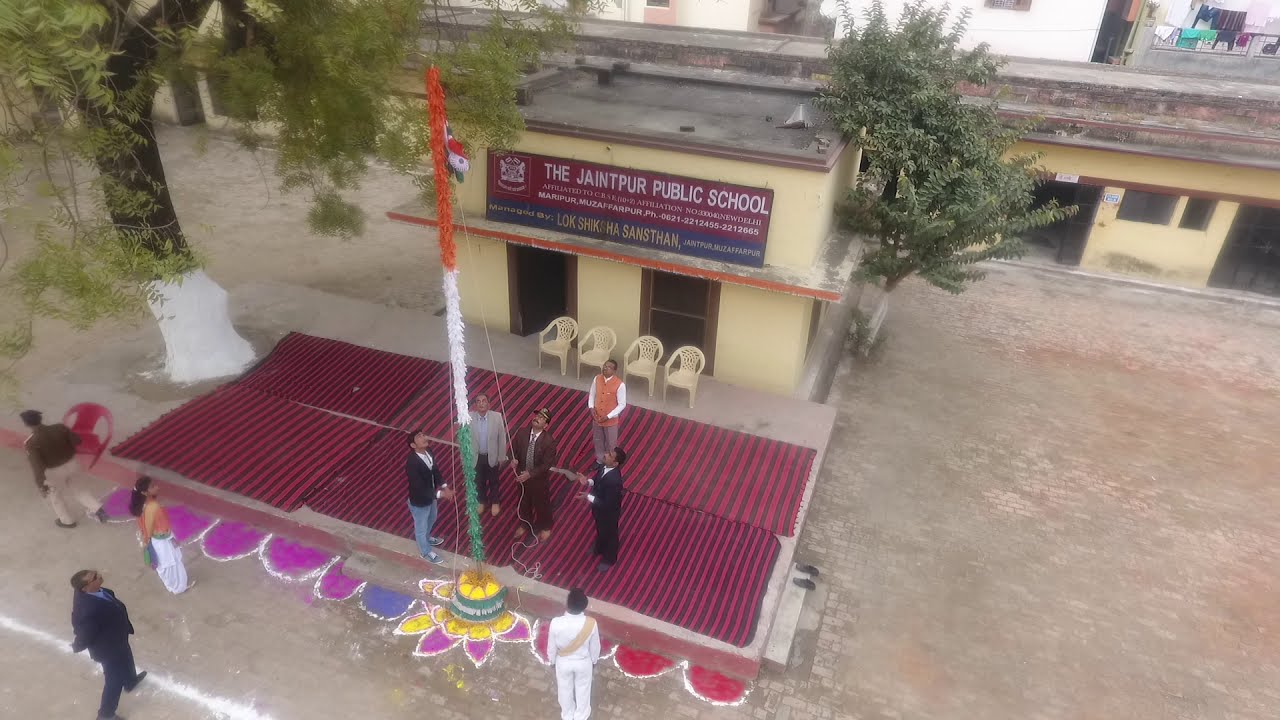In this image, we are in the courtyard of Jaintpur Public School in India. The focus is on a group of people standing on red and black striped mats around a flagpole, which is positioned towards the bottom left of the image. They are raising a colorful flag with green, white, and orange sections, and some yellow at the bottom. The schoolhouse behind them is a small, yellow cement building with a gray and light yellow facade, accented with an orange lining. Atop the schoolhouse is a dark red banner with white lettering that reads "Jaintpur Public School," accompanied by a blue banner with yellow lettering. Surrounding the scene are various objects: a tree with a brown trunk and green leaves located towards the northwest of the flagpole, and a line of tan plastic chairs positioned behind the mats. The ground around the courtyard is a mix of light gray bricks and dirt. The visual is captured from a somewhat aerial view, emphasizing the vibrant, multicultural setting and the communal effort in raising the flag.